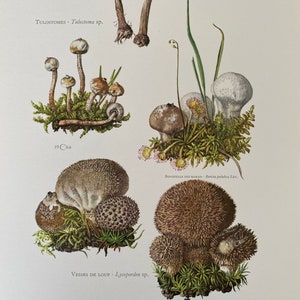The image depicts a set of low-resolution, blurry artworks of various plants and mushrooms against a solid gray background. There are four distinct groups of fungi or plants arranged in the image, each accompanied by illegible black text beneath them. In the bottom right corner, there's a green-leaved plant featuring a large brown bulb surrounded by smaller brownish bulbs. Next to it, a brownish mushroom with spiky, button-like caps emerges from some greenery at its base. To the left, a similar but lighter brown mushroom with less prominent spikes is seen. The top right showcases two white button mushrooms alongside a darker mushroom, all accompanied by foliage. Lastly, to the top left are tall-stemmed fungi with little roots, and next to them, stumpier mushrooms with long stems and white to yellow caps.